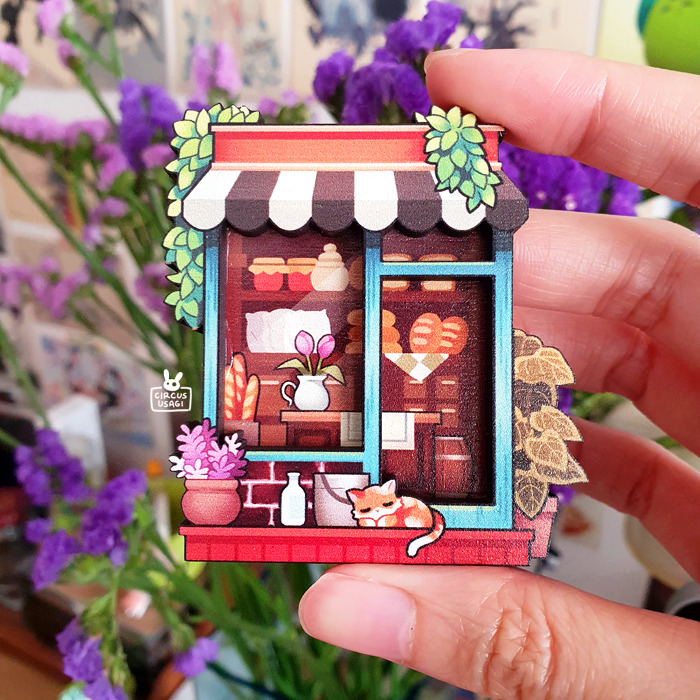In the image, a light-skinned human hand holds a miniature, intricately carved wooden storefront, likely representing a quaint bakery. The miniature shop features a charming brick facade with an orange roof and a black-and-white scalloped awning. The top of the shop is adorned with delicate light green and yellow vines. Inside, the shelves are stocked with loaves of bread, jars of honey, and various containers which might hold cookies or preserves. A white ceramic jug filled with pink tulips stands on an interior table, adding a pop of color within the shop.

On the exterior, a sleeping orange kitten lies beside a white vase filled with white and purple flowers, along with various barrels and a bucket. The storefront is completed with blue trim around the door. The background of the image highlights blurry green stems and purple flowers in different shades, creating a soft, whimsical atmosphere.